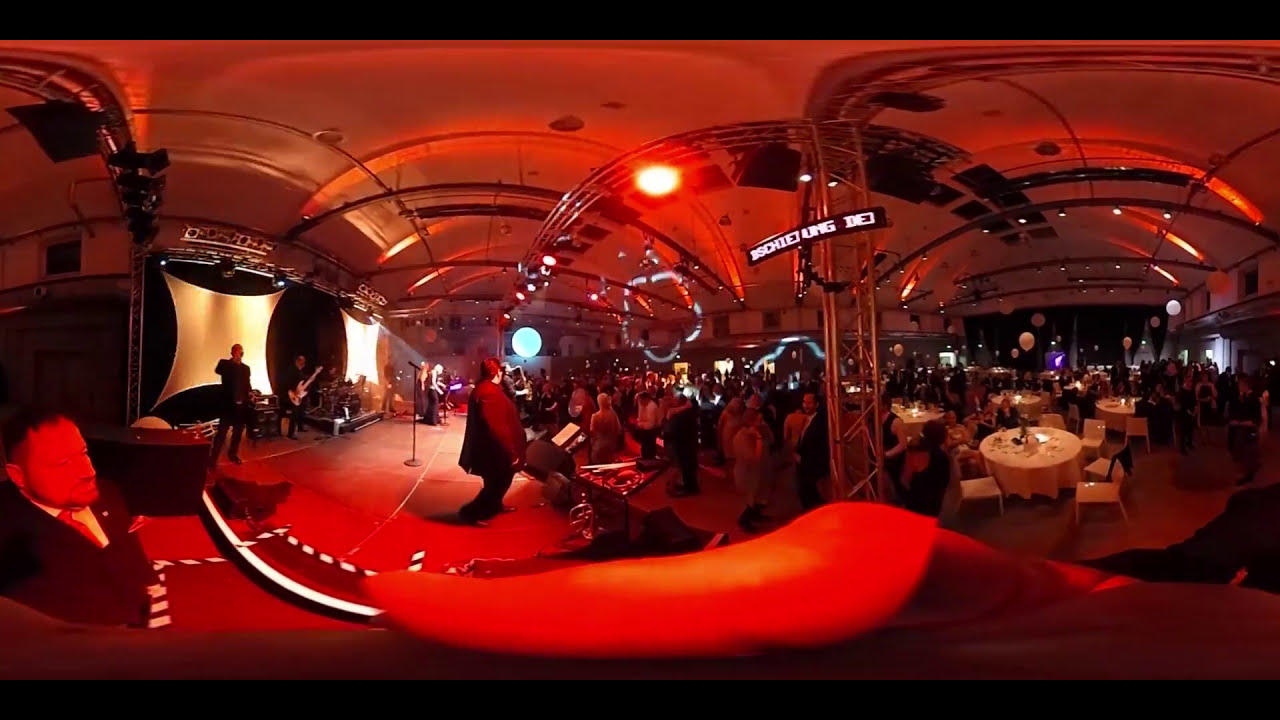This detailed image captures an indoor setting with a unique panoramic perspective, slightly warped by the lens, giving a curved appearance to the top and bottom. The scene is bathed in a red hue, likely due to the lighting, casting a warm, tinted glow over everything. On the far left, partially obstructed, we see a man in a suit with a white shirt and red tie, positioned at the edge of the frame. His thumb and part of his camera are visible, indicating he is the one capturing the image.

Moving further right, there is a stage populated by several people dressed in dark suits, either black or blue. In the foreground on the stage, a singer stands out, while a guitarist with a white guitar is situated towards the back. Centering the image are various tables adorned with white tablecloths, arranged somewhat haphazardly, with groups of well-dressed individuals—men in suits and women in dresses—socializing and enjoying what appears to be a celebration, possibly a wedding or similar event.

A metal framework is visible across the ceiling, enhancing the indoor club-like atmosphere. Balloons can also be spotted among the tables and chairs. To the far right, more attendees are seen mingling in the background, completing the picture of a lively and festive gathering.